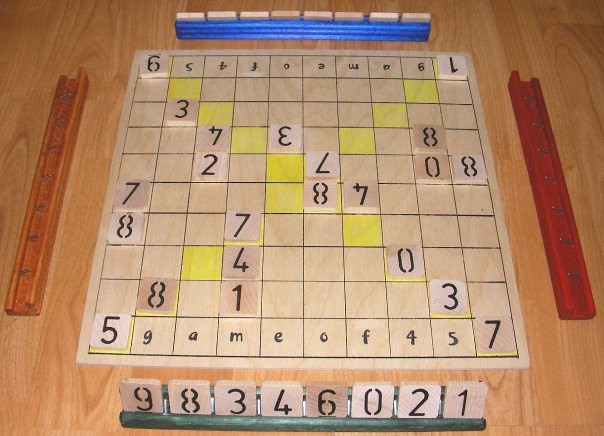The image is a color photograph in landscape orientation depicting a unique, Scrabble-like game in progress, played with numbers instead of letters. The game board is centered on a light pine-colored wooden table with a beach-toned grain running vertically from top to bottom. The square game board itself, which says "Game of 45" on each end, features a grid of equal black-printed squares and is bordered by a slender edge.

Surrounding the board are four wooden holders, one on each side, with raised profiles along their longest lengths. The holder closest to the viewer is painted dark green, the one directly opposite is royal blue, the left holder is light brown, and the right one is cherry red. Each holder is designed to accommodate the square pine-colored tiles, which have black numbers stamped on them. Currently, the green and blue holders have tiles in place, while the brown and red holders are empty. 

Several numbered tiles have already been placed on the board, including prominent numbers like five in the lower left corner, seven in the lower right corner, six in the upper left corner (which might also be read as a nine), and one in the upper right corner. The gameplay objective appears to be to arrange these tiles so their sums approach to or match the number 45, indicating a scoring mechanism central to the game's rules.

The scene presents a richly detailed snapshot of a seemingly homemade game that accommodates four players, evoking curiosity and inviting engagement through its colorful and methodically organized components.